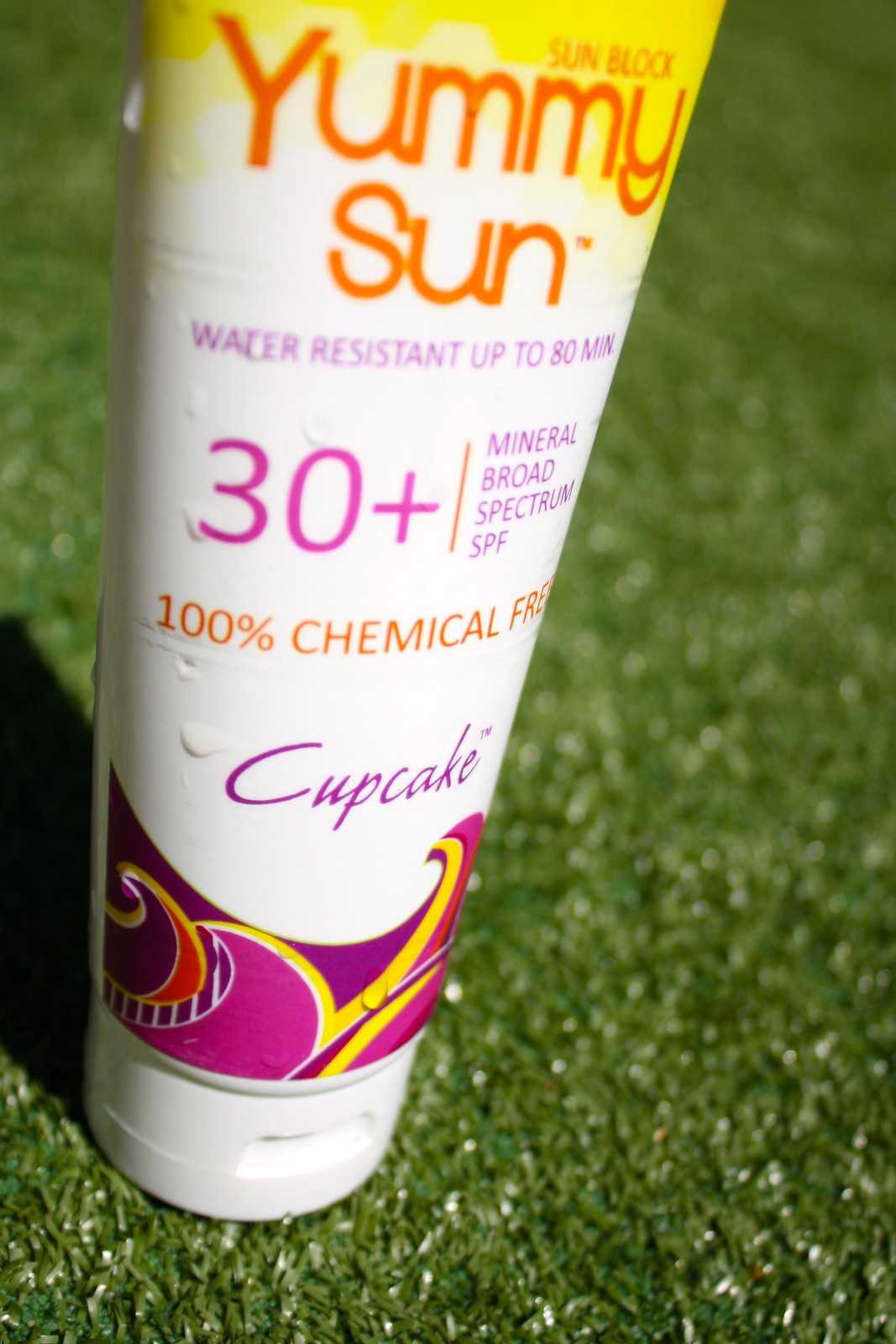This vertically aligned rectangular close-up image captures a container of sunscreen called "Yummy Sun" placed on grass, likely artificial turf, under a sunny sky. The tube features a white cap and a predominantly white body with sections of orange, yellow, purple, and red. The very top portion of the tube is yellow, adorned with "Yummy Sun" written in large orange letters. Just above this, "SUNBLOCK" is printed in all caps in smaller letters. Below the brand name, "water-resistant up to 80 minutes" is inscribed in purple, all caps font. There is a prominent "30+" in purple next to a vertical line separating it from the text "mineral broad spectrum SPF." Further down, "100% chemical free" is highlighted in orange, and beneath that, the term "cupcake" indicates the flavor in purple text. The bottom part of the tube showcases some elaborate swirled designs against a purple background. The bottle is sitting upright on the grass, its bottom part being white with some purple patterns where the sunscreen would be dispensed.